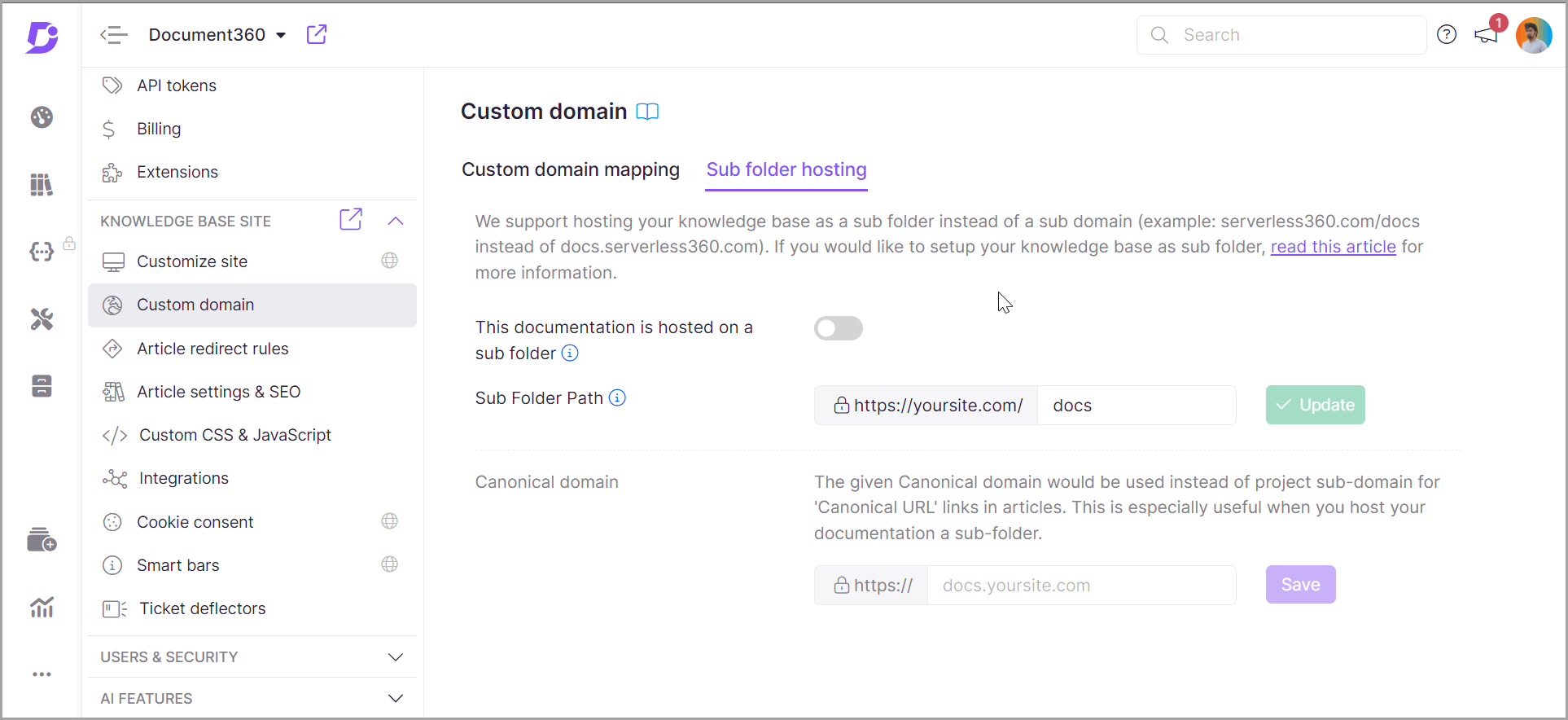The image depicts a rectangular interface with a detailed layout. At the top left corner is a gray border, featuring a slanted purple block 'D' beside a circle with a white outline. Below the circle is a timer icon rendered in gray. Directly beneath that, three book icons appear, with the rightmost book slanted as if leaning on the adjacent two books.

Following this, two gray brackets with three dots between them are positioned, and towards the upper right section lies a light gray padlock. Just below this, a crossed screwdriver and wrench icon is prominently displayed, with the screwdriver oriented leftward and the wrench extending to the right.

Beneath the crossed tools, a gray icon of a bureau is visible. A considerable gap equivalent to three fingers' width separates this section from a cascading folder icon, also gray, with a circular plus sign at the bottom right. Adjacent to the folder, a bar graph topped with a line graph, both in gray, is seen.

Further down, at the bottom left corner of the interface, three dots are lined up horizontally. Toward the right, a menu structure begins at the top left with an arrowhead pointing left and three horizontal bars, with the middle bar longer than the top and bottom bars. To the right of this icon, in black text, "document360" is displayed without a space, accompanied by a downward-pointing black arrowhead.